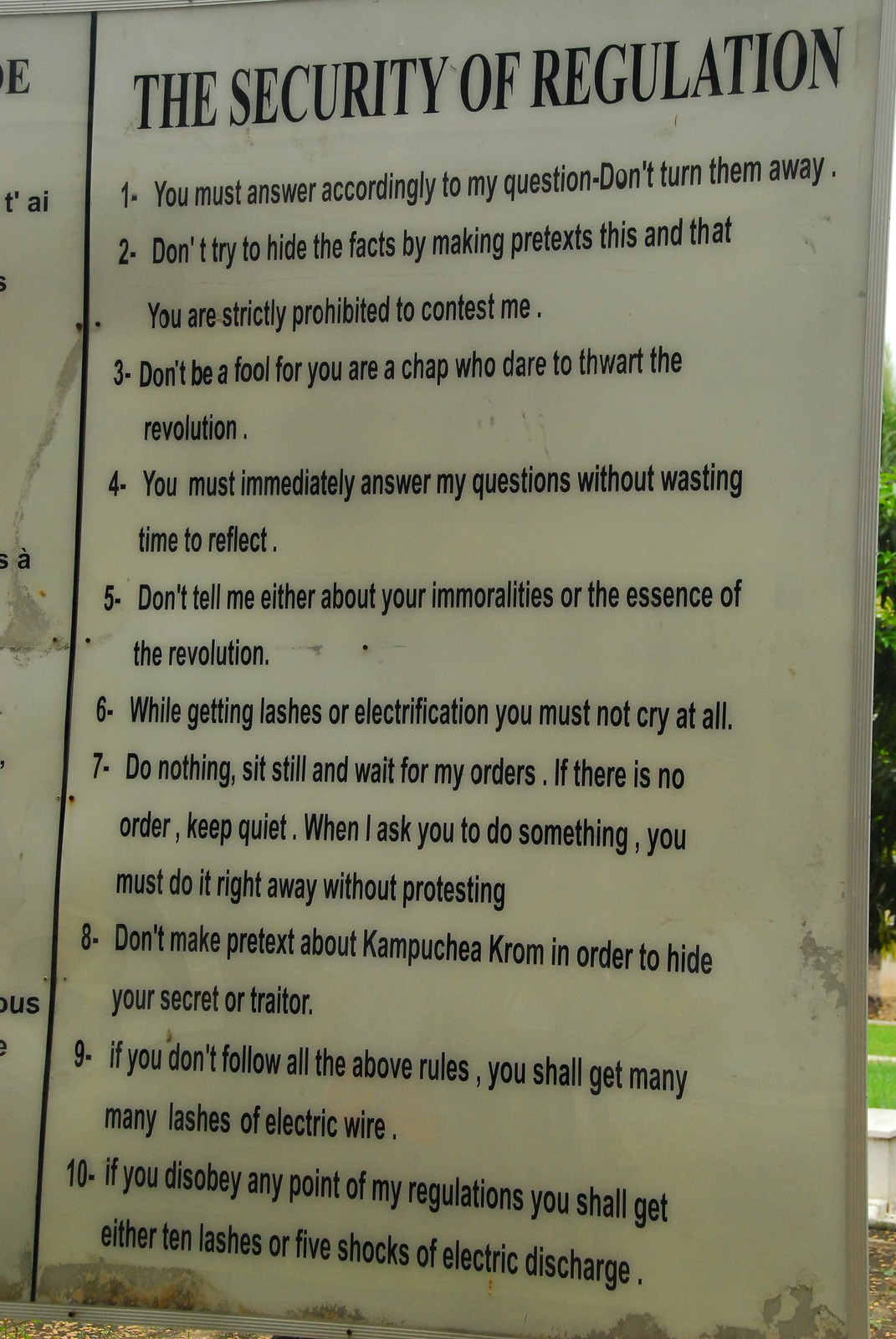This black-and-white photograph depicts a weathered and water-spotted sign announcing "The Security of Regulation" in large black capital letters at the top. The aged and dirty appearance of the sign, with its background faded to an almost greenish hue, indicates its significant age and exposure to the elements. Below the title, the sign lists ten strict rules, each numbered from 1 to 10. The rules outline a series of commands and prohibitions, emphasizing compliance and immediate obedience. Specific directives include answering questions promptly, not making excuses, and maintaining silence unless ordered otherwise. The harsh consequences for disobedience are highlighted, such as receiving multiple lashes or electric shocks. This descriptive content, combined with the sign's deteriorated condition and authoritarian tone, suggests it originates from a historical period or region known for strict and oppressive governance.